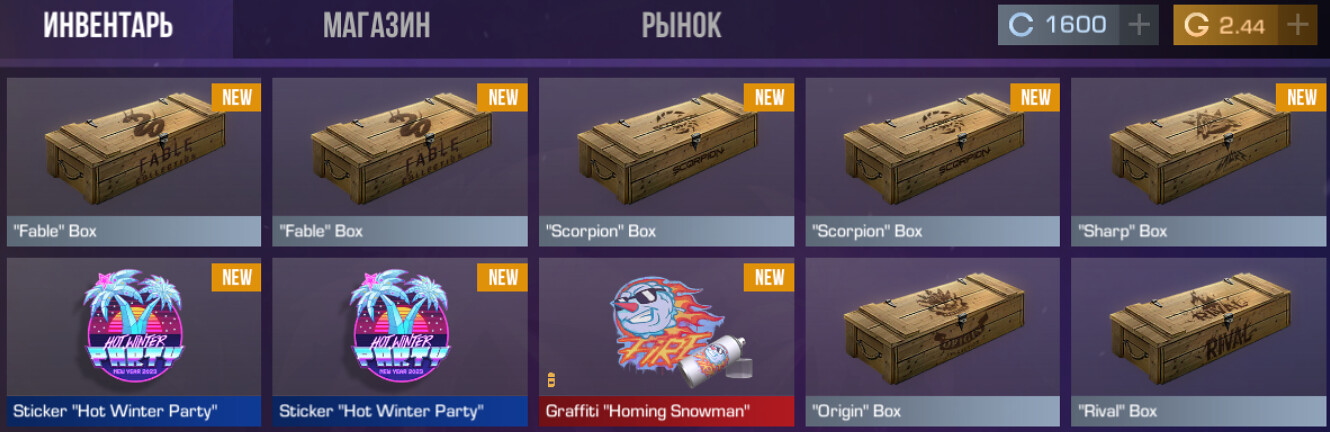This image is a screenshot from a video game store or asset shop, exhibiting a dark purple rectangular interface with ten purchasable items organized into two rows of five. The text at the top appears to be in Russian, featuring three tabs, and the store interface displays two different types of currencies: one blue with an icon 'C' showing $1600 and another yellow-gold with an icon 'G' showing $2.44. Each item in the interface is labeled in English, indicating the contents of wooden crates and other purchasable assets. These labels include "fable box," "scorpion box," "origin box," "rival box," among others. Apart from the wooden crates, three items appear to be stickers or some kind of visual art for the game, with labels such as "sticker," and "hot winter party." Overall, the screenshot provides a detailed look at a typical microtransaction store within a video game, showcasing various collectible and purchasable in-game items.